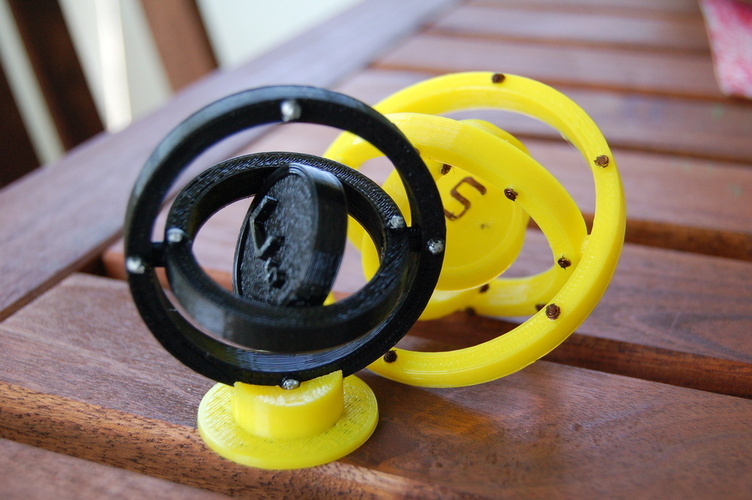The photograph showcases an outdoor setting, likely a backyard or patio, featuring a weathered wooden table or bench with spaced slats forming a horizontal base. The focal point of the image is two distinct 3D-printed objects resembling gyroscopes or directional globes. These objects, both featuring circular discs encased by rotatable rings, appear to serve an unknown function. The one on the left is black, seemingly sturdier, with a letter "C" visibly marked on its central coin-like disc. The one on the right is yellow, smoother in texture, and has an "S" inscribed on its central disc. The background includes a glimpse of a chair and a purse, adding hints of a casual, lived-in outdoor space.